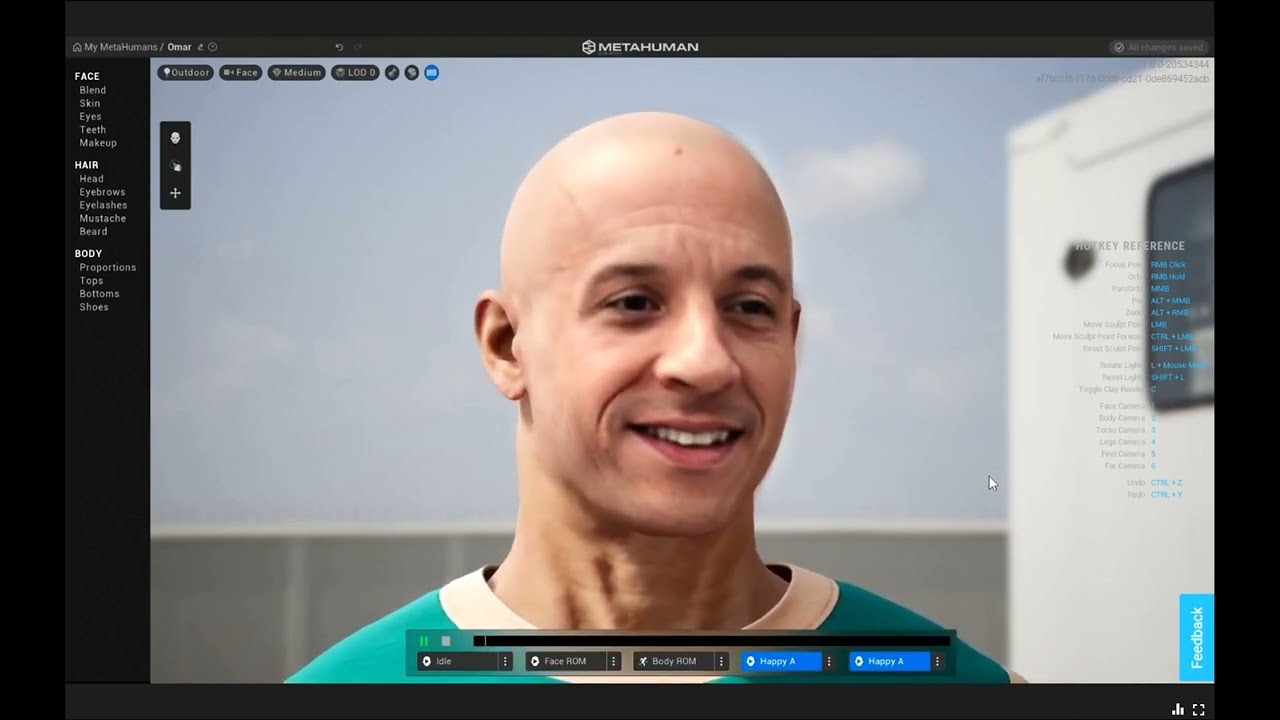This landscape-oriented screenshot appears to be from a digital application or programming database, featuring a sleek, rectangular interface with a black background. The frame includes vertical black borders on the left and right, with grayish bands at the top and bottom. 

At the upper portion of the screen, a home icon precedes the username or program title "MyMetaHuman," displayed prominently. To the right of this, a white icon and the name "MetaHuman" are visible, indicating the name of the application or tool in use.

On the left-hand side, a vertical navigation bar is present, suggesting customization options. This menu includes categories such as 'Face,' 'Hair,' and 'Body,' each presumably expanding to offer further customization features.

The central focus of the image is a detailed, lifelike depiction of a bald man resembling Vin Diesel. The AI-generated character, looking slightly to his left (viewer's right), exudes a friendly demeanor with a broad smile, displaying his teeth. He's dressed in a green shirt with a collar that appears to be a yellowish-tan color, enhancing the realism of the virtual character. This screenshot likely illustrates a customizable avatar being modified within the application, highlighting the software's capabilities in human-like digital representation.